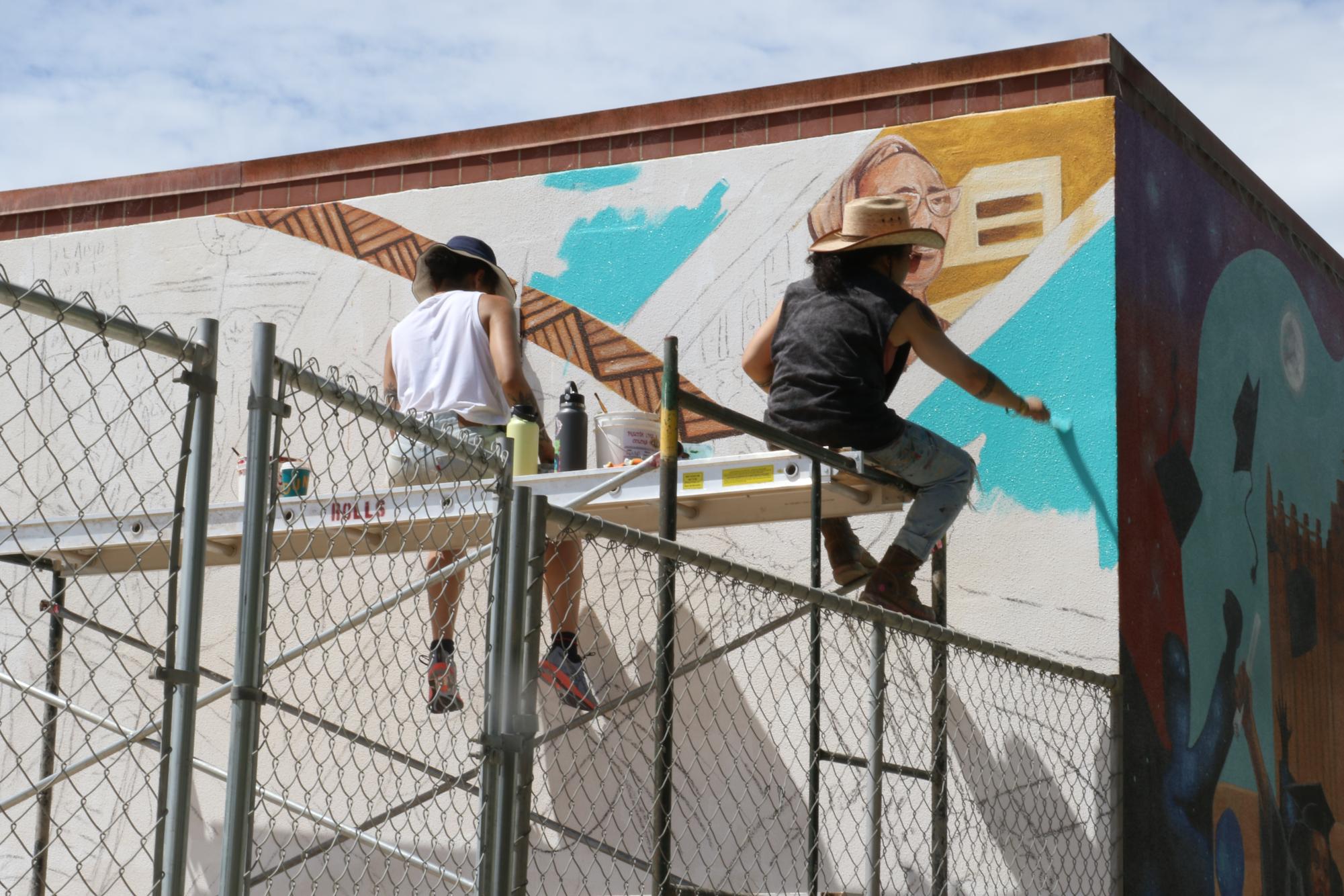In the photograph, two men are seated on top of metal scaffolding, working diligently on painting an elaborate mural on the corner of a building. The men, both wearing wide-brimmed hats and safety vests, are distinguished by their attire—the man on the left sports a white tank top with short jeans and tennis shoes, while the man on the right wears a black shirt and long jeans paired with a cowboy hat. The mural, adorned with an array of colors from light cream to dark brown, aqua blue, and golden yellow, is designed with intricate geometric shapes and varying textures. This work-in-progress spans a building approximately 20 feet tall and 40 feet long, and the section they're working on is set within a fenced-off area. The right side of the building features the finished portion of the mural, showcasing elements like a blue sky and a detailed man's face, whereas the left side still shows a predominantly cream base, awaiting further artistic touches. Despite the simplicity of the unpainted side, the colorful and textured mural on the right hints at the eventual grandeur of the entire wall.